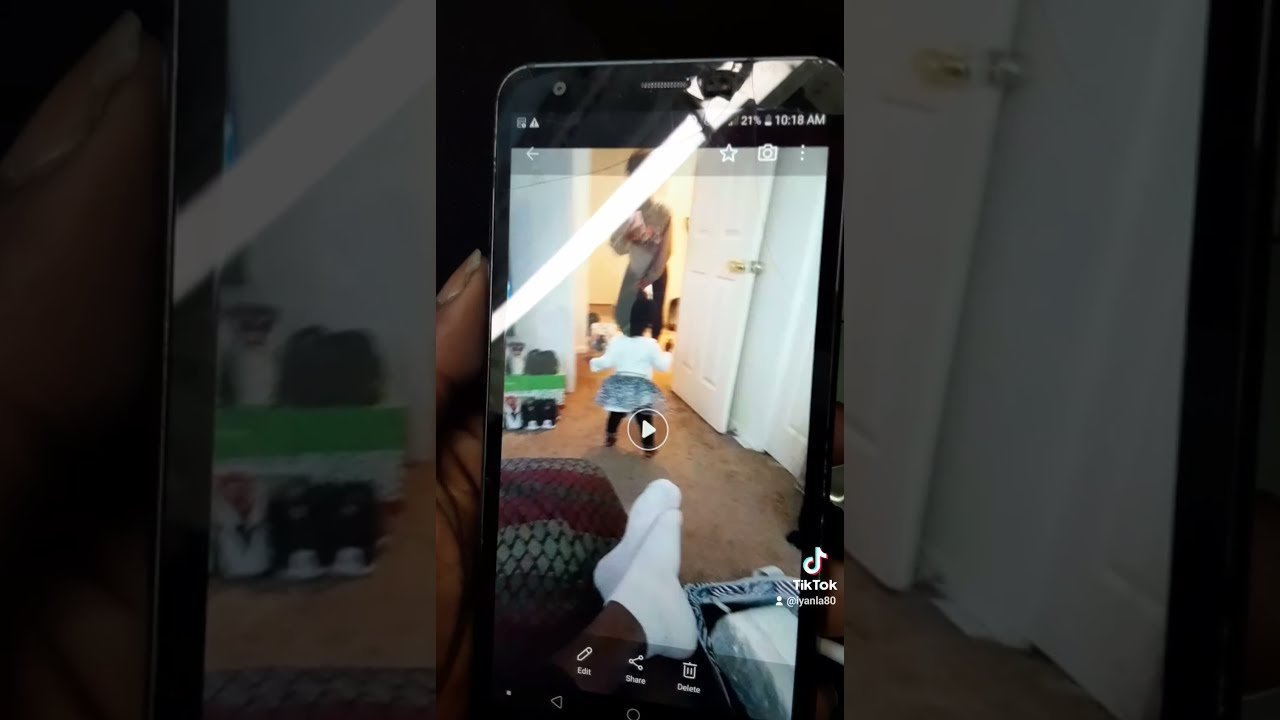This detailed image captures a vertical, portrait-oriented photograph of a smartphone screen displaying a TikTok video. The main image reveals a young person, possibly in their 30s, standing in the doorway of their bedroom. The individual is dressed in black pants and a sweatshirt. In the background, the room is detailed with a TV to the left, a shelf stacked with shoes, a brown laundry basket with white socks near it, and a toddler playing with toys on the floor. The smartphone is held by a hand, with the TikTok logo visible in the bottom right corner. The whole scene is set against a zoomed-in, darkened background that mirrors the central photograph, contributing to a distinct photographic style that emphasizes the realism of a cell phone capture.